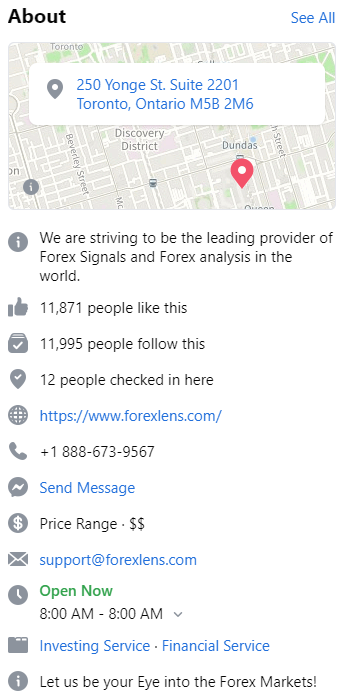The image displays information on a mobile device screen providing details about a business. In the top left corner, "About" is written in bold black letters, while in the top right corner, "See All" is in blue letters, appearing as a clickable link. 

Below this heading is a street map with an inset detail. Overlaid on the map is a white rectangle, indicating a specific location: "250 Yonge Street, Suite 2201, Toronto, Ontario, M5B2M6." A red location pin, represented by an inverted teardrop shape with a white dot, marks this address on the map.

Below the map, there are various details about the business:

- An information icon (a white "i" in a grey circle) accompanies the text: "We are striving to be the leading provider of FOREX signals and Forex analysis in the world."
- A thumbs-up icon indicates: "11,871 people like this."
- A suitcase icon with a checkmark shows: "11,995 people follow this."
- A location icon with a checkmark notes: "12 people checked in here."
- A globe icon leads to a clickable link: "https://www.forexlens.com."
- A telephone receiver icon lists the contact number: "+1-888-673-9567."
- A speech bubble icon with the text "Send Message" in blue suggests a clickable chat function.
- A circle icon with a dollar sign indicates the price range with two dollar signs ($$), suggesting a mid-range pricing.
- An envelope icon provides an email address in blue (also a clickable link): "support@forexlens.com."
- A clock icon in green reads "Open Now," with operating hours stated as "8 AM to 8 AM," suggesting 24/7 availability (though this could be a typo meant to read "8 AM to 8 PM").
- A file icon in blue (clickable) links to "Investing Service" and "Financial Services."
- An eye icon with the text: "Let us be your eye into the forex markets!"

This detailed caption summarizes the mobile device display, accurately conveying the business information, clickable links, and visual elements for a comprehensive user understanding.